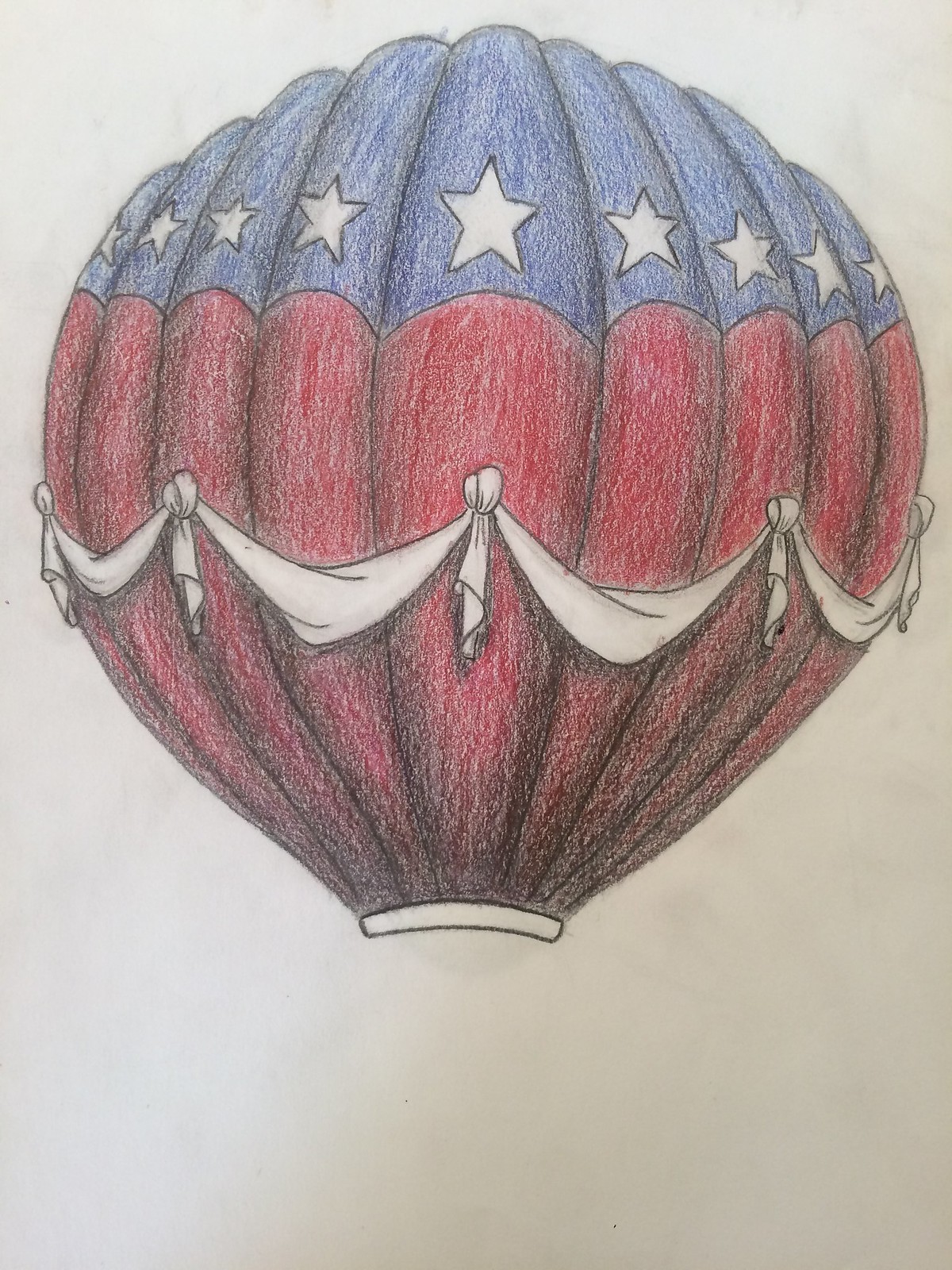The image depicts a detailed hand-drawn illustration of the upper section of a hot air balloon on white drawing paper, which has some black smudges likely from pencil shavings. The balloon's top third is shaded in dark blue, adorned with white, five-pointed stars of varying sizes to suggest depth. These stars are surrounded by the dark blue background. The bottom two-thirds of the balloon transitions into a rich red hue that darkens towards the bottom, enhancing its three-dimensional appearance. Intermittently encircling this red section is a white ribbon resembling a handkerchief, tied and draped in a crescent pattern around the balloon, connecting every other panel. Each segment of the balloon is partitioned by black diagonal lines, creating a sense of depth and structure. The overall image is in portrait orientation and focuses solely on the balloon, omitting the basket typically found at the base.